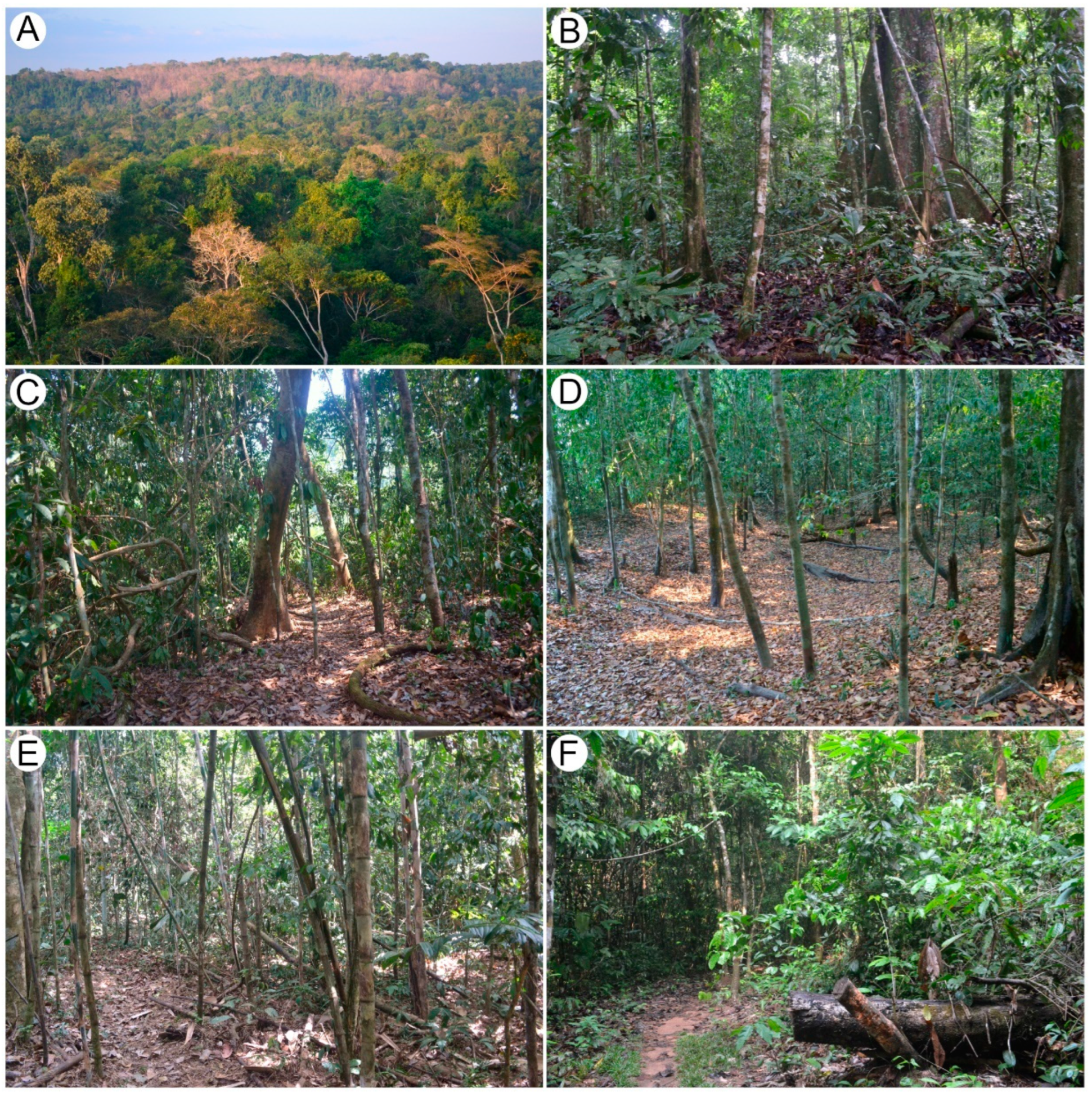This image is a sextych composed of six smaller images labeled A through F, each capturing different aspects of a forest. Image A, in the top left, presents an aerial view of a forest canopy, showcasing a diverse mix of green and brown trees spread across a hillside. Image B, the top center section, offers an interior view of a densely wooded area with a lush green underbrush. Moving to image C, the middle left section, the scene encapsulates a similar thick forest but includes a well-trodden dirt path winding through it. Image D, in the middle right, depicts a less densely packed forest with a bare floor predominantly covered with dead leaves. Image E, at the bottom left, shows a tangle of mostly leafless and small dead trees scattered throughout the area. Finally, image F on the bottom right features another dense forest with a small brown trail and a noticeable fallen log. Each image, whether showing a jungle-like canopy or ground-level views of varied vegetations and trails, collectively captures the different facets of a possibly singular wooded location.